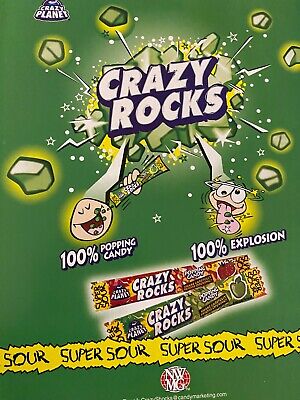The advertisement for Crazy Rocks Popping Candy features a vibrant green background with the product name "Crazy Rocks" prominently displayed in white letters at the center top. Behind the text, green crystal-like rocks appear to be exploding with scattered stars, sparks, and small rock fragments, creating a dynamic and energetic visual. 

Below the product name are two whimsical cartoon characters indulging in the candy. The character on the left has their eyes closed in delight, savoring the candy pouring into their mouth, while the character on the right appears comically disoriented with stars swirling around their head, eyes crossed, and tongue out, showcasing green rocks on it. This detail highlights the candy's intense and playful nature, enhanced by the accompanying phrases "100% Popping Candy" and "100% Explosion".

Towards the lower part of the image, there are two packets of Crazy Rocks candy. The red-yellow packaging, adorned with a small strawberry, indicates a strawberry flavor, while the green-yellow packaging with a small apple suggests a green apple flavor. Both packages prominently display the product name "Crazy Rocks."

A yellow banner runs across the bottom of the advertisement with the phrase "Super Sour" repeated in bold black letters, emphasizing the candy's sourness. In the lower left and right corners, additional branding elements feature a red globe with "NWMG" and the logo "Crazy Planet" in blue text, suggesting the producers of this lively and nostalgic candy.